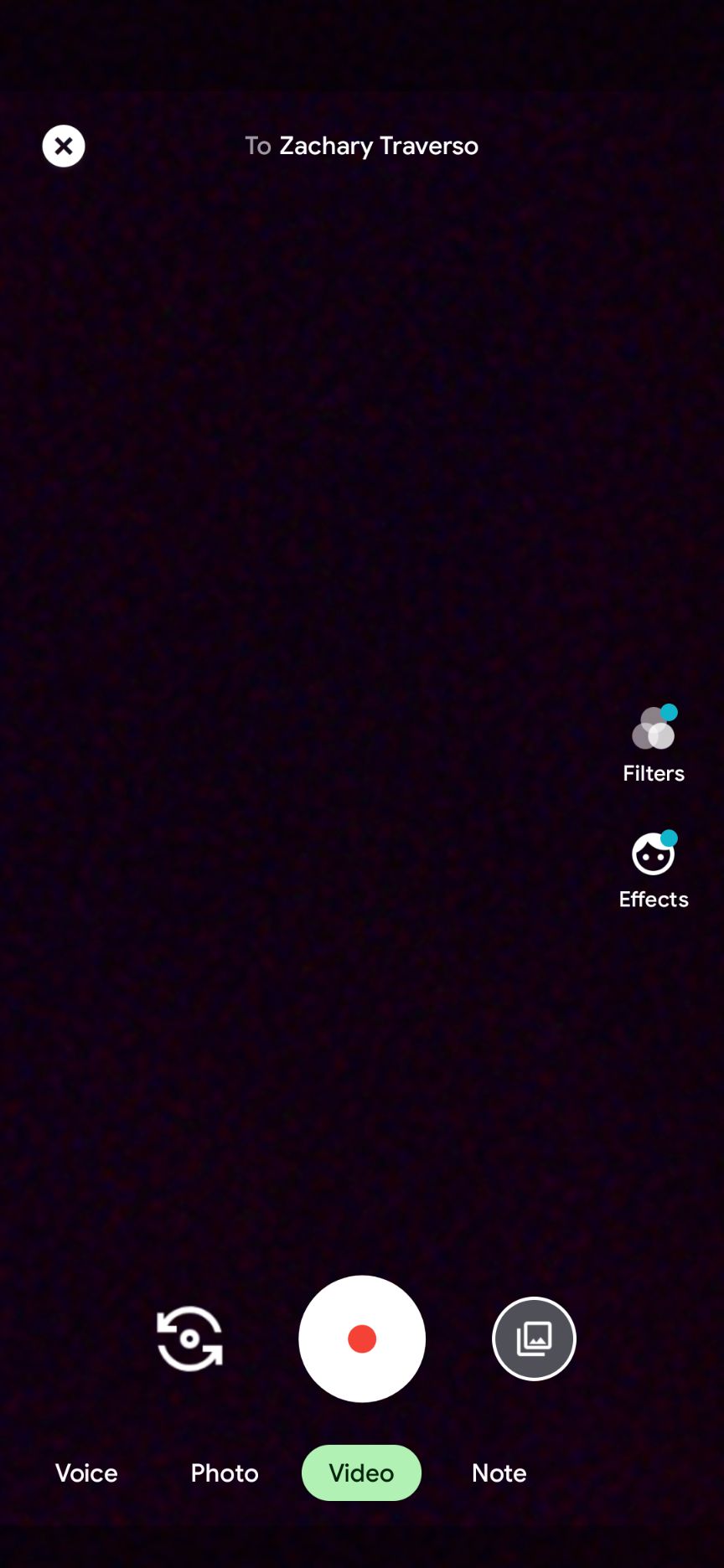A screenshot showcases a predominantly black interface, punctuated by a few distinct elements. At the center is a solid white circle featuring a black 'X' in its middle. Directly above this is a black filter bar, which offers various filter options: three in grey, and one in blue. Adjacent to the filter bar, a small icon displays a blue dot with the label "Effects." Beneath these elements, the interface provides options for replaying or recording content. At the bottom of the screen, a navigation menu presents choices labeled "Voice," "Photo," "Video," and "Note," with "Video" currently highlighted. At the top of the screen, the name "Zachary Traversa" is prominently displayed.